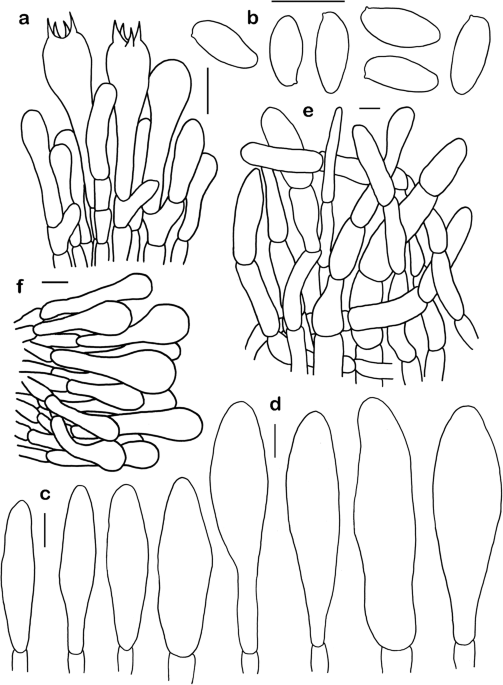This black and white hand-drawn diagram, possibly rendered in pencil or pen, illustrates a series of six labeled figures, A through F, which display various forms of irregularly shaped, Q-tip-like structures. 

- **A:** Features a cluster of elongated, bulb-ended stems with some spiky tops, resembling small plant-like structures tightly grouped together.
- **B:** Depicts a small pile or cluster of six objects that appear similar to flower petals or beans.
- **C:** Shows a group of elongated and irregular shapes, aligned vertically and resembling oblong Q-tips or the stretched top of a kitchen knife.
- **D:** Presents a larger version of the shapes seen in C, comparable to a larger dinner knife, still retaining the Q-tip-like appearance.
- **E:** Displays a jumble of intertwined, segmented blobs that suggest the skeletons of finger bones or the flanges of a plant.
- **F:** Illustrates these Q-tip-like structures lying horizontally, similar to algae or growing microbes.

The overall composition is a simple yet detailed line drawing, providing a complex view of various stages or perspectives of these mysterious structures.